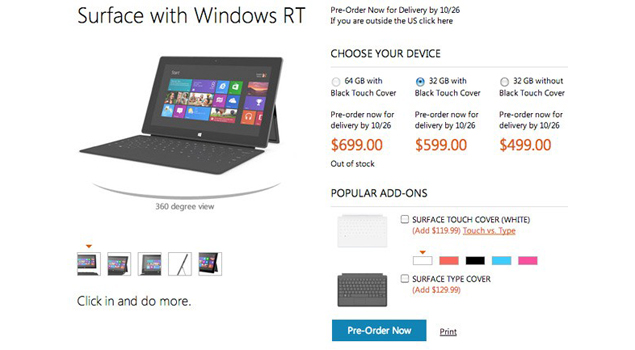This is a detailed screenshot of a web page selling a Windows laptop. The background of the page is white with black text, interspersed with various colored numbers and icons for pricing and menu items.

At the top of the page, in large black text, are the words "Service with Windows RT," followed by a prompt to "Pre-order now for delivery by 10/26." Below this, there's a notification for international users: "If you are outside of the US, click here."

A subheading reads "Choose your device," under which there are three menu options to order the laptop. On the left-hand column of the webpage, there is an image of the laptop. The laptop features a colorful screen showcasing Windows icons and a sleek, slim design. The screen appears to be between 13 to 15 inches, with a keyboard placed in front of the display.

To the right of this image, there are three selectable options for purchasing the laptop. The middle option is highlighted with a blue radio button, indicating it has been selected. This option describes a 32GB model with a black touch cover, priced at $599, with delivery guaranteed by October 26th (10/26).

The other two options are priced at $699 and $499, presenting different configurations. Additionally, there are several customizable add-ons, such as a surface touch cover available in various colors (fuchsia, black, aqua, and pink) and a surface type cover, which acts as a keypad cover.

At the bottom of these options, there is a "Pre-order now" button, concluding the detailed presentation on the web page.